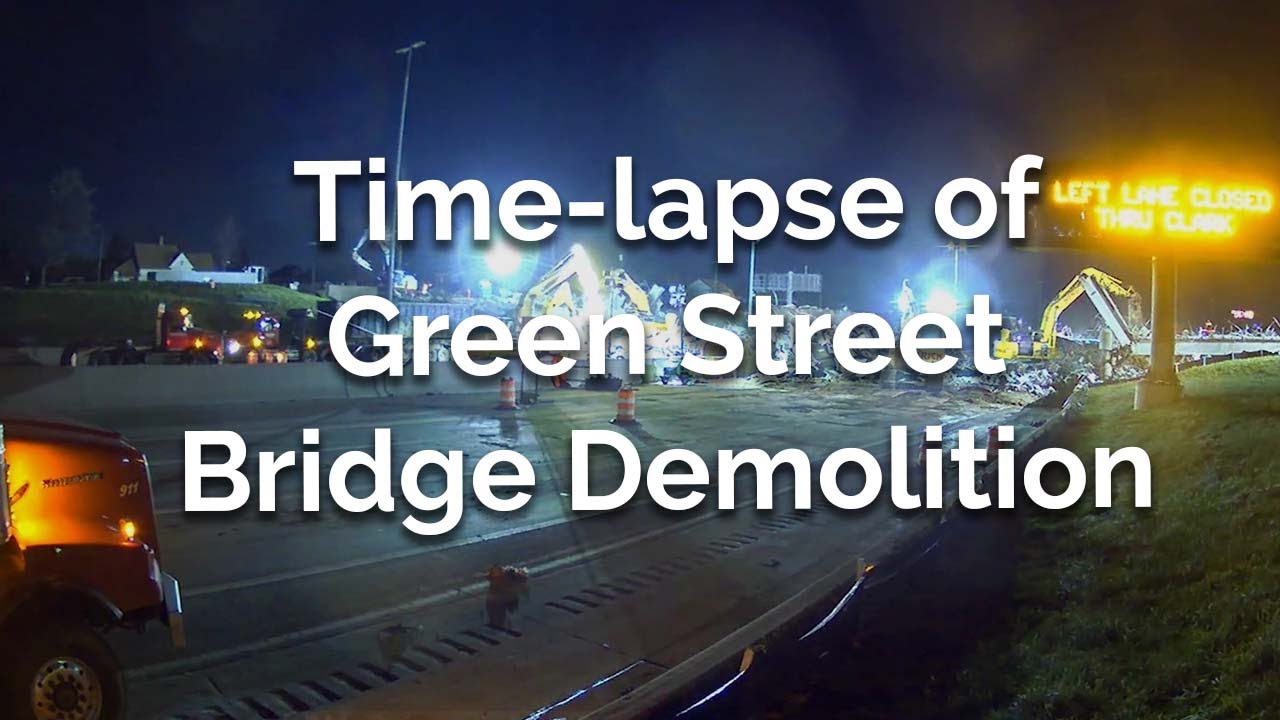The image displays a nighttime scene of construction equipment set against the backdrop of a bridge demolition, accompanied by white text with a subtle drop shadow that reads "time lapse of Green Street bridge demolition." The illuminated area features various heavy machinery, including cranes and the partially visible front end of a yellow truck in the lower left corner. On the right side of the scene, a digital sign glows with the message "left lane closed," though the bottom portion is too overexposed to decipher completely. The surroundings include bright construction lights, orange traffic cylinders, and grass on the right side. A single white house with a brown roof is visible in the upper left, contrasting with the industrial activity below. The overall impression is one of an introductory frame for a time-lapse video capturing the dramatic nighttime demolition of the Green Street Bridge.